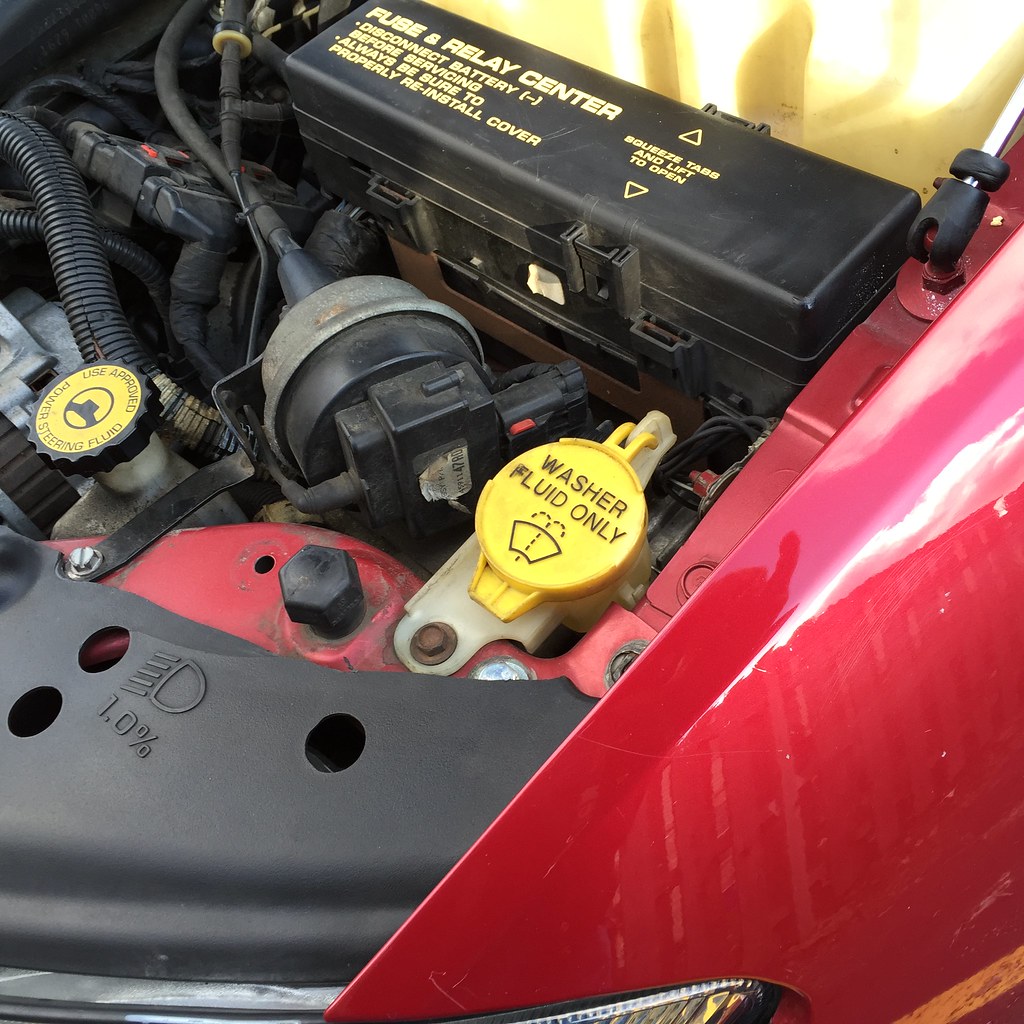This image displays the interior of a red vehicle's engine compartment with several key components clearly visible. The red front panel of the car creates a diagonal line in the lower right corner of the image. Centrally located is a yellow cap that indicates "Washer Fluid Only," accompanied by the washer fluid icon. To its left, we find a similar yellow cap for approved power steering fluid with a yellow sticker for easy identification. Multiple black hoses run through the compartment, connecting various elements. In the upper right section, there's a black fuse box marked with yellow text, "Fuse and Relay Center," including critical instructions: "Disconnect battery (negative) before servicing" and warnings to properly reinstall the cover. Visible further are parts of the headlight at the very bottom center and the hinge of the hood. Overall, the image showcases a well-organized engine bay with various ports and components easily identifiable against the field of red and black.